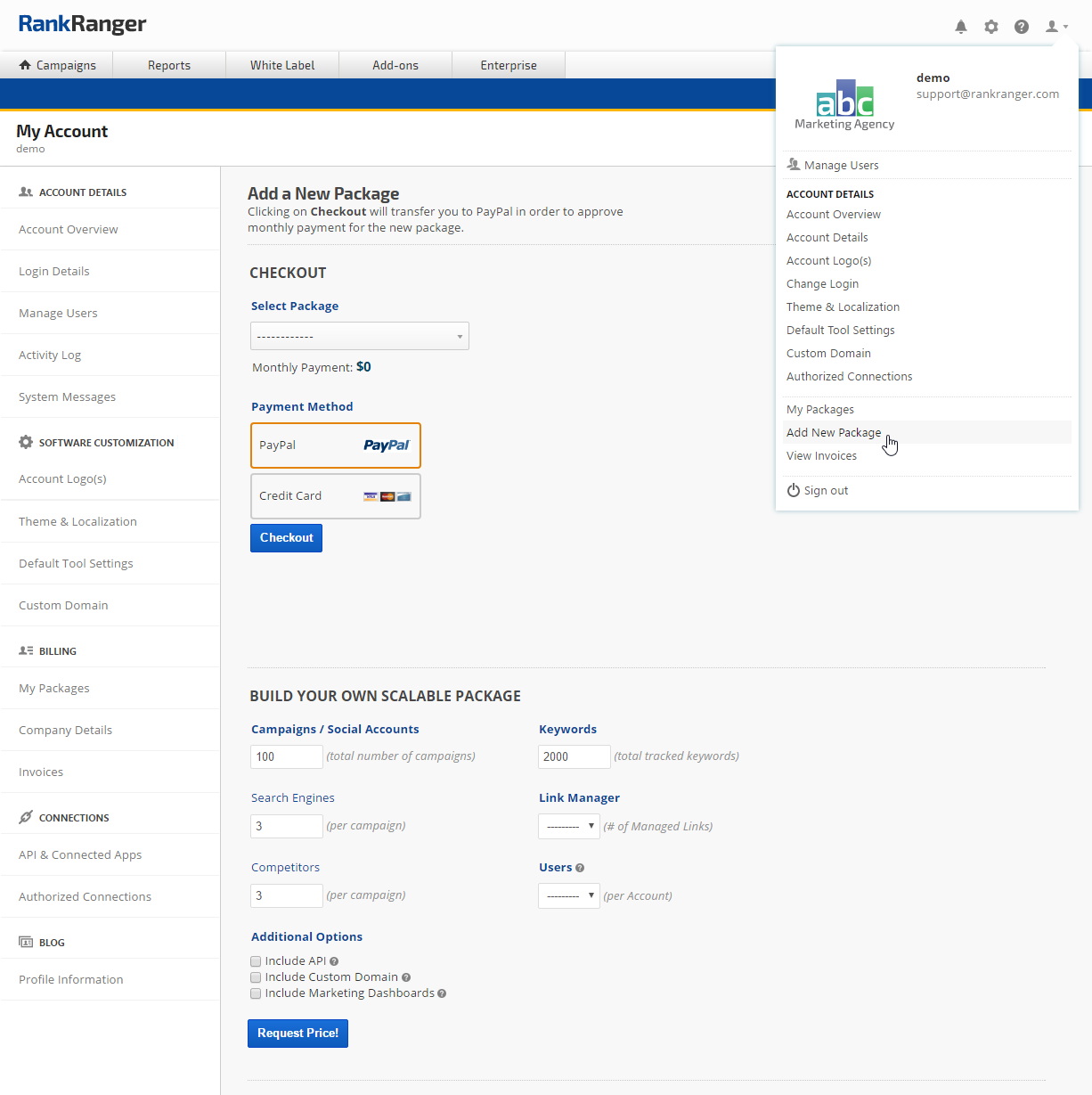The image shows the interface of RankRanger, a comprehensive SEO and marketing analytics tool. At the top of the interface, the RankRanger logo is prominently displayed. On the upper right-hand side, tabs for Profile, Settings, Notifications, and Help are clearly visible. The cursor is hovering over the Profile tab, triggering a drop-down menu labeled "ABC Marketing Agency" and a demo indicator.

In the drop-down, several options are available: Manage Users, Account Overview, Account Details, Account Logos, Change Login, Theme and Location, Default Tool Settings, Custom Domain, Authorized Connections, and various package management options like My Packages, Add New Package, View Invoices, and Sign Out. The left-hand sidebar mirrors these options and additionally includes tabs for Connections, Billing, and Software.

Under the packages section, users can select different payment methods such as PayPal and credit card. Upon choosing a package, the interface shows the monthly payment details and allows users to build customizable packages based on search engines, keywords, competitors, and other options. To request a price, users can click the blue "Request a Price" button located below the package customization options.